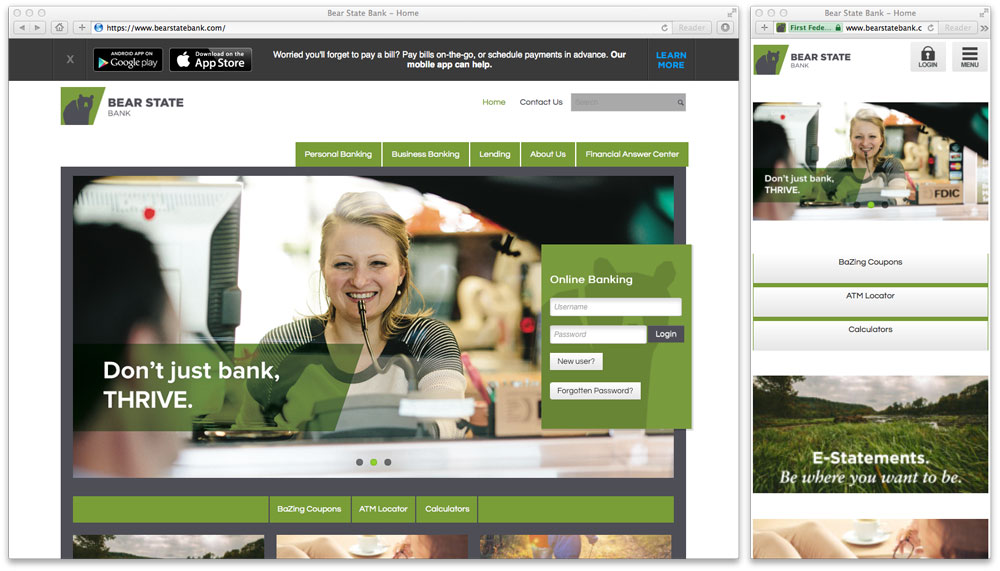**Detailed Caption for Bear State Bank Home Page Image:**

The Bear State Bank home page features a prominent gray header at the top that reads "Bear State Bank Home." Below this, the branding section prominently displays a logo: a green shape with an irregular contour, wider at the top than the bottom, and a black bear inside it beside the text "Bear State Bank." Directly underneath, a navigation menu with green tabs and white text offers options such as Personal Banking, Business Banking, Lending, About Us, and Financial Advisory Center.

Dominating the central section of the page is an image of a blonde woman in a white, gray, and black striped shirt, where the stripes on her arms are narrower than those on the front. She holds a microphone to her mouth, suggesting she is providing customer assistance. Adjacent to this, a green rectangle catches the viewer's eye with the motivational text "Don't Just Bank, Thrive."

To the right of the central image is a login section for Online Banking framed in a clear square. Here, users are prompted to enter their username and password to log in, with links for "New User" and "Forgotten Password" for further assistance.

Lower on the page, a gray rectangle spans the width beneath the main sections, and nested within it is a green rectangle containing three smaller white rectangles. Each of these smaller rectangles holds text for different utilities: "Coupons," "ATM Locator," and "Calculators."

At the bottom, partially visible photos form an intriguing strip. The leftmost image shows clouds and trees, the center image reveals more clouds, and the third image appears to be a map, all contributing to the overall aesthetic of the web page.